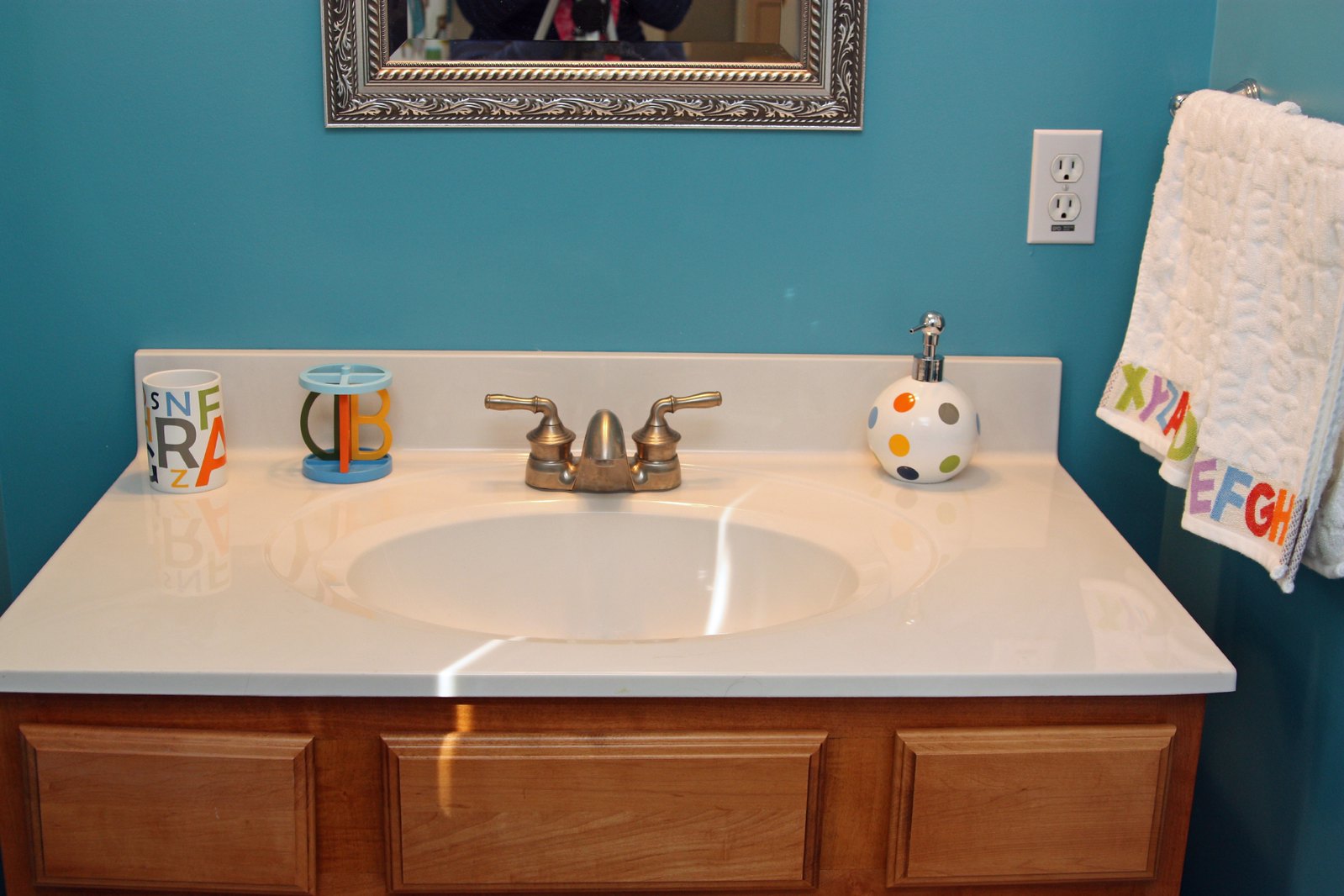In this vibrant bathroom scene, the walls are painted a striking turquoise, creating a fresh and lively atmosphere. The medium wood vanity stands out with its rich tones and features three intricate decorative panels just below the pristine, bright white cultured marble countertop. The sink matches the countertop in its dazzling white hue and is complemented by gold-colored fixtures, with separate hot and cold faucets adding a touch of classic elegance.

Adorning the sink area are a variety of colorful accessories, adding playful elements to the space. A cup embellished with multicolored letters in orange, green, blue, and gray takes center stage, accompanied by a modern toothbrush holder that mirrors the same vibrant palette. Additionally, a liquid soap dispenser with whimsical polka dots in matching colors around its round white base completes the cheerful ensemble, making this bathroom both functional and visually engaging.